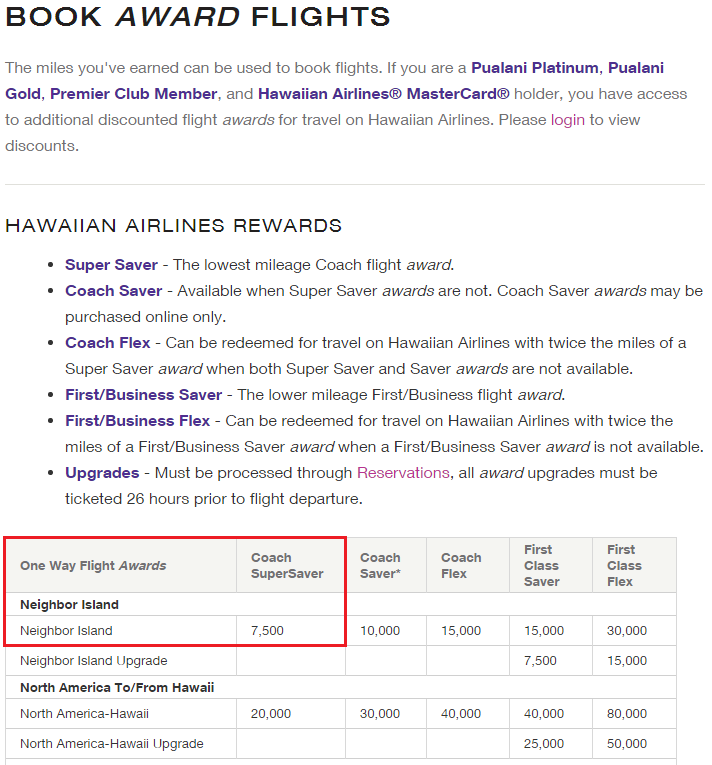The image features a predominantly white background with detailed information about Hawaiian Airlines' award flights and rewards program. 

At the top left corner, "Book Award Flights" is prominently displayed in black letters. Below it, smaller gray text reads, "The miles you've earned can be used to book flights. If you are a Palani Platinum, Palani Gold, Premier Club Member, and Hawaiian Airlines MasterCard holder, you have access to additional discounted flight awards for travel on Hawaiian Airlines. Please log in to view discounts." Notably, "Palani Platinum," "Palani Gold," "Premier Club Member," and "Hawaiian Airlines MasterCard" are highlighted in purple, while "log in" is marked in pink. 

Following this, a fine gray line separates the introductory text from the subsequent section titled "Hawaiian Airlines Rewards" in black. Six reward categories are outlined, each with a purple title accompanied by a gray description:

1. **Super Saver**: Indicated by a purple dot, it is identified as the lowest mileage coach flight award.
2. **Coach Saver**: Available when Super Saver awards are not, these awards can only be purchased online.
3. **Coach Flex**: Redeemable for travel on Hawaiian Airlines with twice the miles of a Super Saver award when both Super Saver and Saver awards are unavailable.
4. **First Business Saver**: The lower mileage award for First Business Class flights.
5. **First Business Flex**: Can be redeemed for travel on Hawaiian Airlines with twice the miles of a First Business Saver award when a First Business Saver award is not available.
6. **Upgrades**: Must be processed through reservations, with all award upgrades needing to be ticketed 24 hours prior to flight departures. "Reservation" is highlighted in pink.

Additionally, there's a chart outlining one-way flight awards under the following categories: Coach Super Saver, Coach Saver, Coach Flex, First Class Saver, and First Class Flex. The chart details the mileage required for various flight routes:

- **Neighbor Island flights and upgrades**: Coach Super Saver costs 7,500 miles, with specific numbers listed for Coach Saver, Coach Flex, First Class Saver, and First Class Flex awards.
- **North America to Hawaii**: Detailed mile requirements for each award type, including upgrades.

A bold red box highlights the "One-way flight awards, Coach Super Saver, all the way down to Neighbor Island," emphasizing the 7,500-mile requirement. The chart systematically presents mileage information for Neighbor Island, Neighbor Island upgrade, North America from Hawaii, North America-Hawaii, and North America-Hawaii upgrade categories, covering both economy and first-class options.